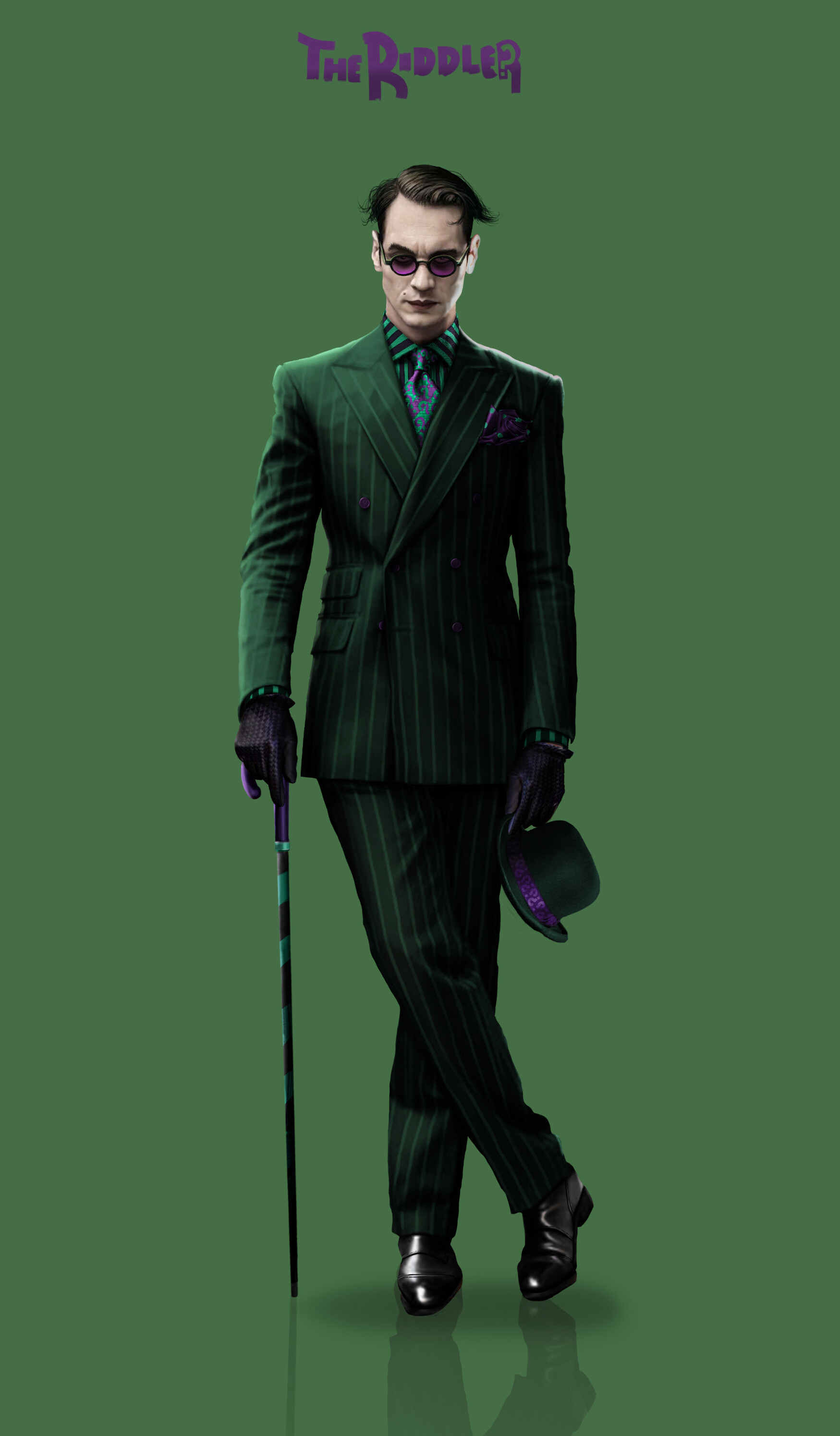This detailed movie poster illustration features The Riddler, a character from the Batman series. The background is a sinister forest green, providing an eerie atmosphere. The Riddler is stylishly dressed in an emerald green pinstripe suit, complemented by a purple and green tie. His attire is accentuated with purple gloves, a square pocket in purple, and shiny black dress shoes with legs crossed. His left hand holds a green and purple top hat with a purple ribbon around the rim, while his right hand is propped on a cane that has green and purple stripes, resembling a candy cane pattern. The Riddler's face is very pale with coiffed hair and purple-tinted sunglasses perched on his head. The title of the movie, "The Riddler," is displayed in stylized purple font that incorporates The Riddler's iconic question mark into the "R". This 3D styled digital illustration also includes a faint reflection of The Riddler on the ground, adding depth to the sinister ambiance of the poster, making it a captivating visual for a movie advertisement.